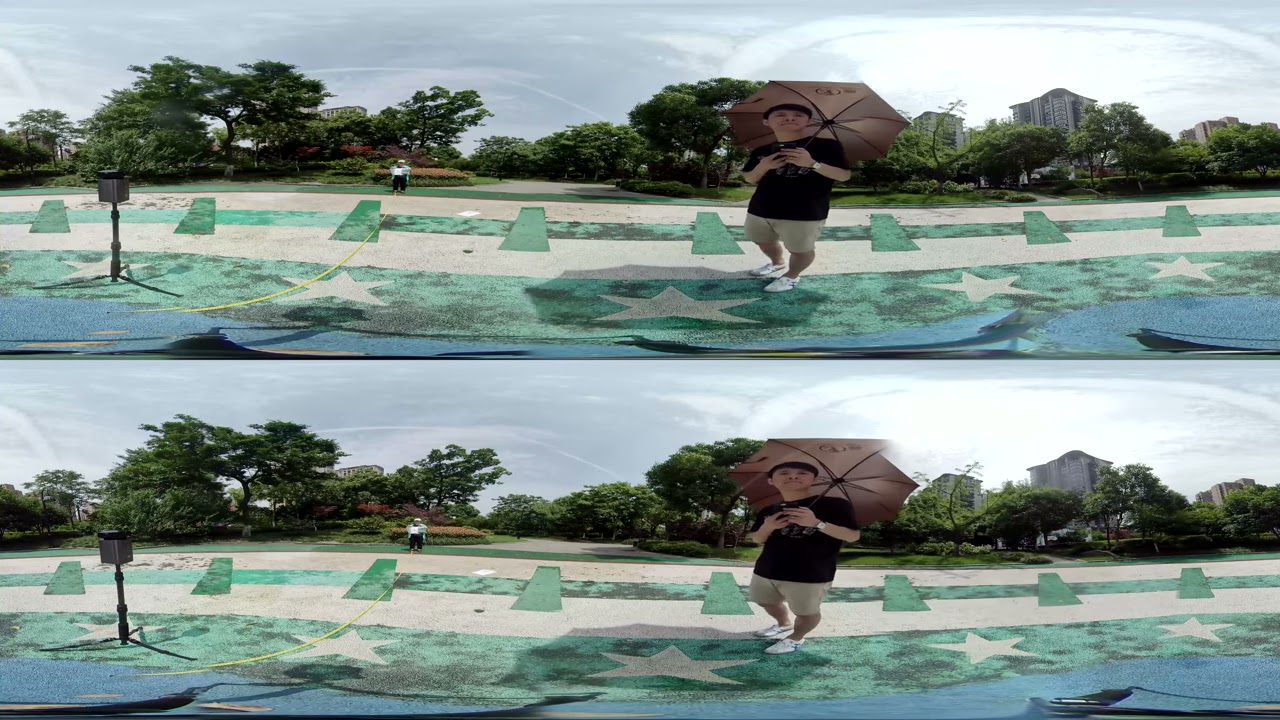The image features two identical stacked photographs taken outdoors during the daytime, with a light gray sky scattered with white clouds. In the center-right of the photograph is a young Asian man, likely in his early 20s, walking from the right side to the left side. He is dressed in a black short-sleeved t-shirt, tan shorts, white sneakers, and a silver watch on his left wrist. He holds a brown umbrella over his left shoulder. His hands are raised towards his chest, and he gazes upward, over the viewer’s right shoulder. 

The man is walking on a green walkway punctuated with white stars, and his right foot is on a light tan strip of turf while his left foot is on green turf. Below this is a blue band of turf stretching across the image. The layout of the walkway includes a green band with white stars, followed by a white band, and then another green band with vertical stripes, resembling a railroad design. This final green band might be actual grass, extending to the far side of the image.

On the left side of the image is a black rectangular speaker on a stand, with a yellow wire extending upwards. In the background, to the left of center, is another person standing at a distance. This person is wearing a white cap, gray jacket, white shirt, and black pants. The backdrop includes tall green trees, patches of green grass, some buildings on the far right and left sides, and the overall setting suggests a park or garden, perhaps a tourist spot.